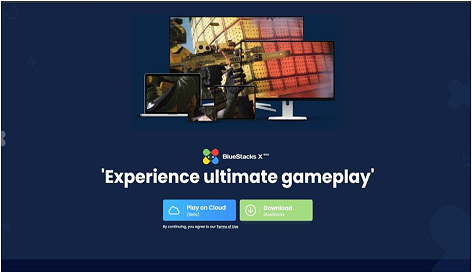**Caption:** "The advertisement features a sleek, navy background that serves as a striking canvas for an array of electronic devices, including a small laptop, a tablet, a regular-sized TV in the far background, and a monitor prominently in the foreground. These devices collectively display a seamless, complete image across their screens, suggesting an integrated visual experience. This setup is branded by Blue Shades X, whose unique logo consists of three colored circles—green at the top left, red to the right, blue underneath, and yellow. The circles converge around an indistinct central shape. Below the logo, a bold tagline reads, 'Experience Ultimate Gameplay,' clearly targeting gaming enthusiasts. The ad further offers interactive options with a blue tab labeled 'Play on Cloud' and a green tab for 'Download,' emphasizing the flexibility and convenience for gamers."